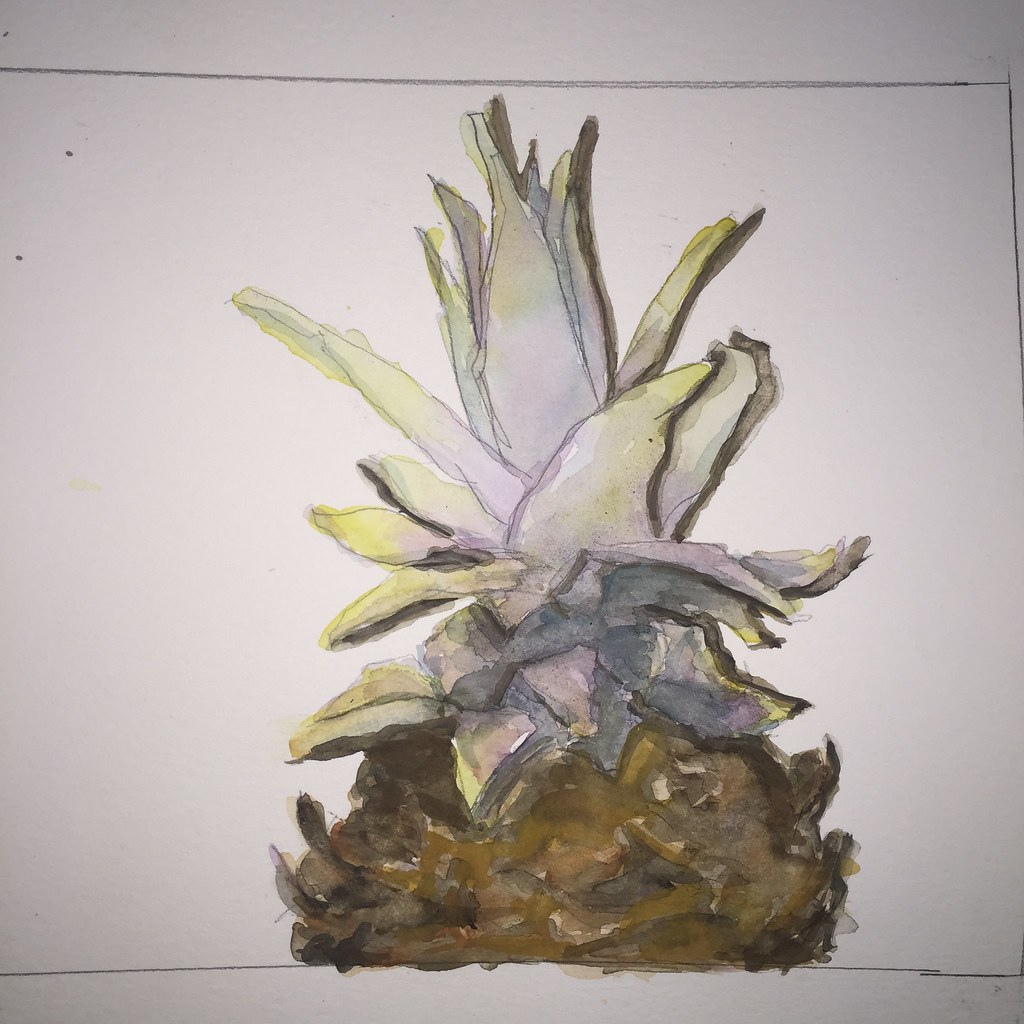The image depicts a hand-drawn and watercolor-painted artwork on sketch pad paper, set against a white background. Framed within a gray square, the focus is on a section of a pineapple top. The lower part of the pineapple is illustrated with sharp, dark to light brown hues that mimic the texture of pineapple bark. The upper part, featuring serrated leaves, is a blend of light green to yellow shades, with touches of gray and purple. The leaves fan out from the center, creating a vivid, spiky crown. The image appears to be a quick, unsigned sketch enriched with watercolors, showcasing a detailed and colorful representation of a pineapple fragment.